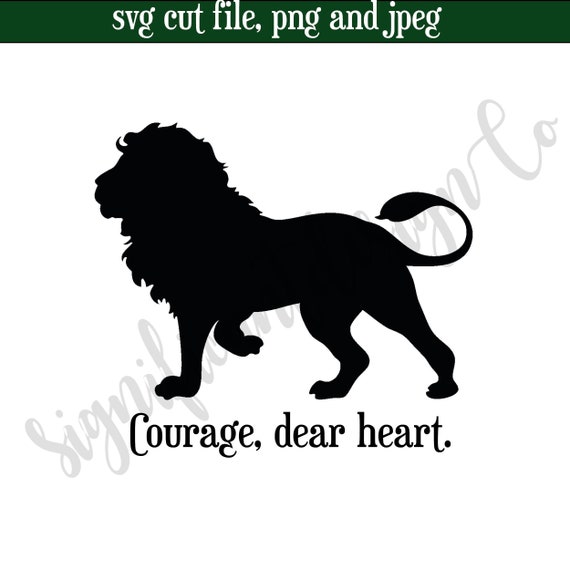This image is a meticulously crafted graphic design illustration featuring a jet-black silhouette of a male lion in profile view, facing left. The lion's distinctive mane, all four legs with one leg slightly curled inward, and his upward-curving tail are clearly defined against a pristine white background. Beneath the lion, in elegant black text, are the words "courage, dear heart." A diagonal gray watermark, written in a script font, spans from the bottom left to the top right of the image, though it clashes with the lion silhouette and is largely unreadable, save for the word 'significant.' At the image's top, a dark green stripe houses white text that reads "SVG cut file, PNG and JPEG," indicating the image formats this design is available in.